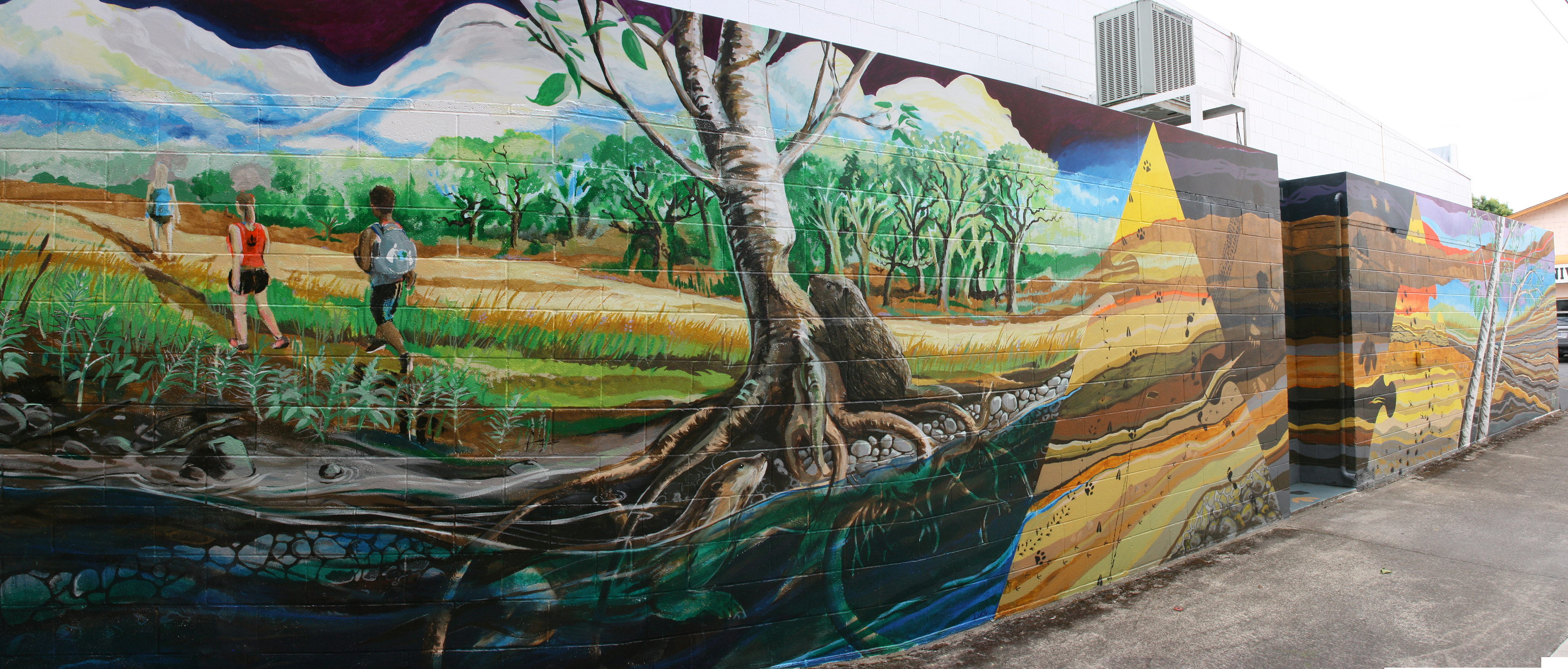The image depicts a vibrant mural painted on the side of an exterior block wall in what seems to be an urban setting, captured on an overcast day with a white sky above. The mural itself is divided into two sections. The section nearest to the camera prominently features three young individuals walking along a narrow pathway, flanked by lush gardens on either side. The figures, depicted from behind, are dressed in distinct attire: the foremost in a short-sleeved blue shirt, followed by another in a red tank top, and the last wearing a gray shirt with what appears to be a backpack. Dominating this part of the mural is a tree resembling a birch, its roots visibly extending into a waterway that runs in front of it, with a beaver gnawing a half-moon shape into its trunk. Beside the tree stands a pyramid, its soil-covered structure leading up to a bright yellow pinnacle. The adjacent section of the mural portrays a serene landscape of trees by a lake, creating a harmonious blend of natural elements across the wall's expanse.